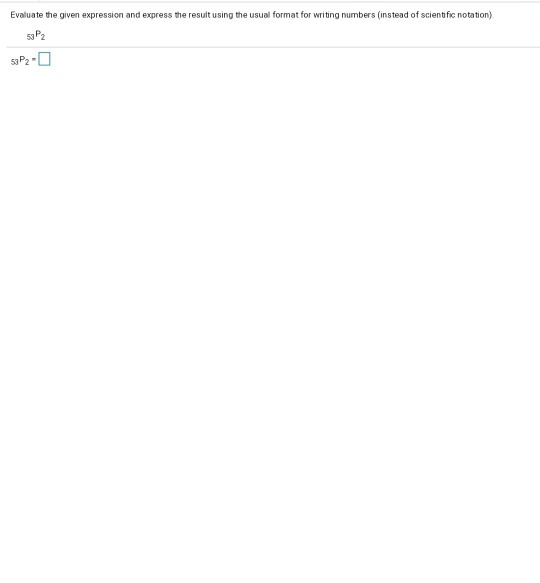The image depicts a screenshot likely taken from an educational assessment tailored for secondary school or university students enrolled in a mathematics course. The central focus is a directive that reads, "Evaluate the given expression and express the result using the usual format for writing numbers instead of scientific notation." Below this instruction, there is a numerical expression featuring "53" in superscript, a capital "P," and a "2" in superscript, indicating a mathematical sequence or permutation. A green box is also present near the expression, possibly meant to highlight or annotate a specific part of the problem. The written instructions are framed by two grey lines, one above and one below, adding structure to the layout. The entire background is white, contributing to a clean and uncluttered appearance. Notably, the image contains no additional pictures, drawings, or illustrations of humans or animals.